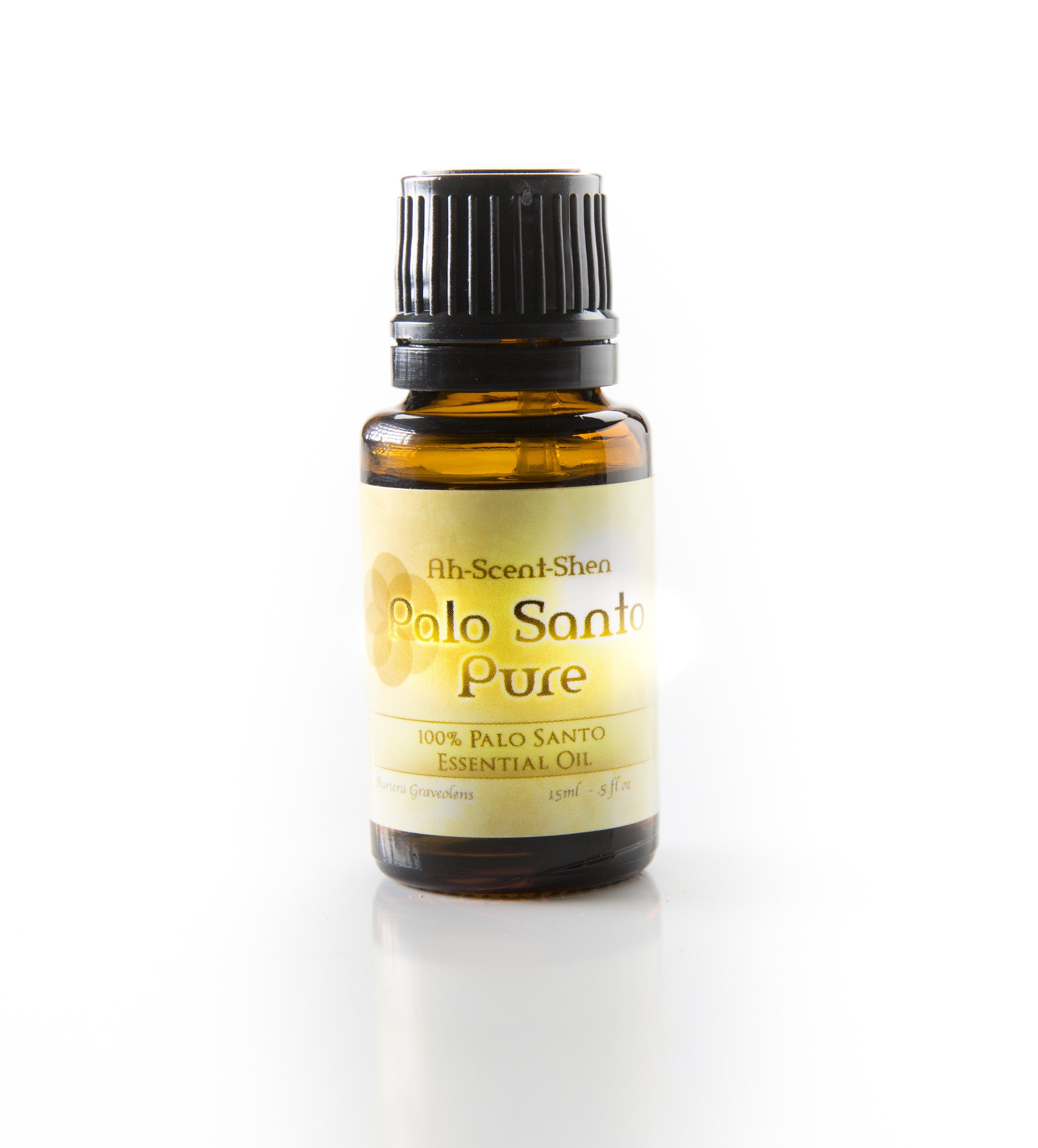This image features a close-up of an amber essential oil bottle with an unopened black cap, featuring a visible safety ring. The bottle is set against a white background, creating a well-lit scene with a subtle shadow beneath the bottle. The label on the bottle is a soft yellow color with darker yellow text. From top to bottom, the label reads "Ascension - Scent Shen" followed by "Palo Santo Pure", "100% Palo Santo Essential Oil", and at the bottom left, "Graveo Leons", with "15ml - 50 FL" on the bottom right. The label is adhered to the bottle, whose hue slightly darkens towards the bottom. The overall presentation highlights the pristine condition of the product.